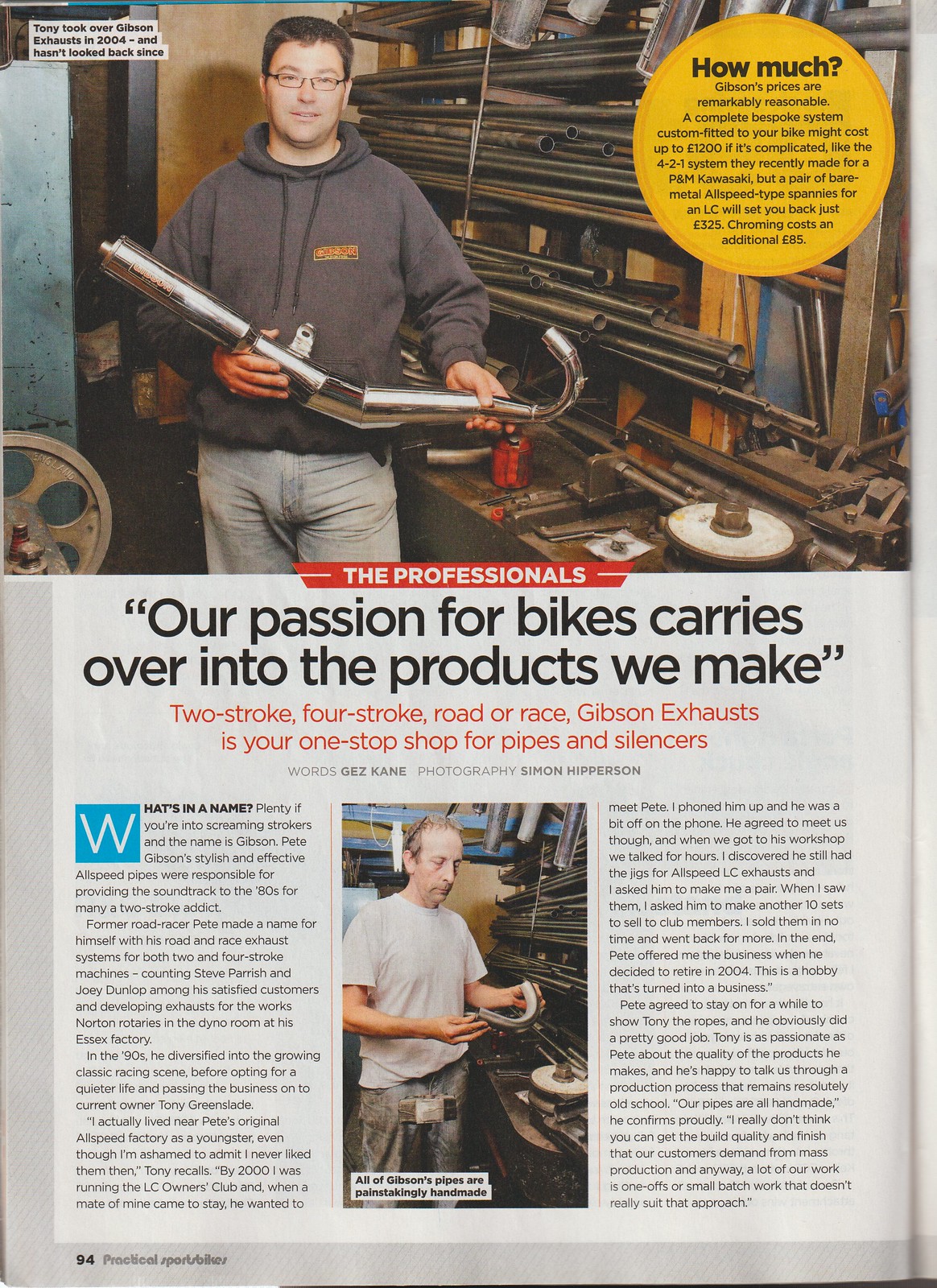The magazine page features an in-depth article about Gibson Exhausts, prominently displaying a photo of a man in a gray sweatshirt and blue jeans holding a shiny metal exhaust pipe, with a backdrop of tools and metal tubing. Above the image, a note mentions that Tony took over Gibson Exhausts in 2004 and has successfully led the company since. To the right, a green circle details the reasonably priced bespoke systems offered by Gibson, with a complete system potentially costing up to £1,200, while a pair of bare metal all-speed pipes for an LC costs around £325, with an additional £85 for chrome. The main article hails Gibson Exhausts as a revered name in the industry, known for their stylish and effective pipes which defined the 80s for many two-stroke enthusiasts. The company’s passion for bikes translates into their high-quality products, catering to both two-stroke and four-stroke engines. Pete, a former road racer, originally made Gibson’s name synonymous with top-tier road and race exhaust systems, counting legends like Steve Parrish and Joey Dunlop among satisfied customers, and even developing exhausts for the Werks Norton rotaries.